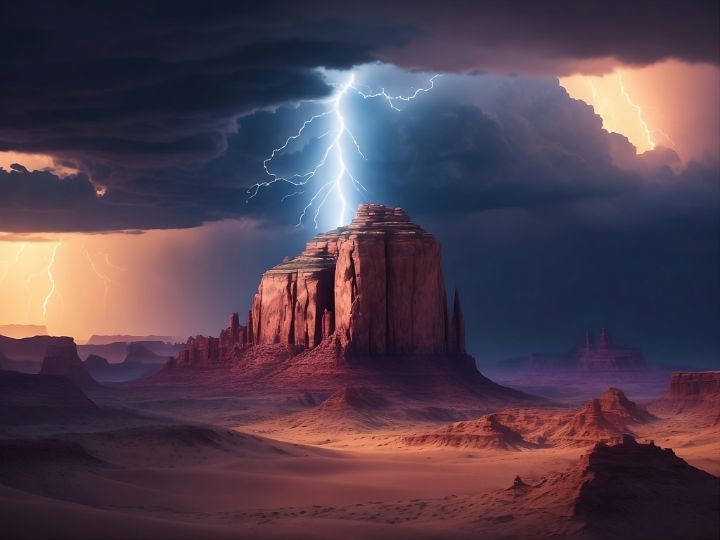The image portrays a captivating and surreal landscape, likely an artistic or illustrative rendition, dominated by deep, intense colors of blue, purple, brown, yellow, and grey. Central to the scene is a towering butte or mountain, characterized by distinct, column-like boulders with hues of brown, red, and purple, suggesting a composition of rock and soil. Surrounding the butte, the ground is rugged and rocky, reminiscent of an alien terrain, though it also evokes earthly desert-like features with its sandy, mountainous area.

The sky above is dark and stormy, filled with thick clouds that cast shadows over the landscape, creating a shadowy atmosphere with minimal light. An almost finished sunset to the right imbues the scene with orange tones, contrasting starkly with the approaching night. A dramatic bolt of lightning strikes the butte, branching out with electric flares and highlighting the dynamic weather at play. Despite the intense natural phenomena, the entire setting feels eerily quiet and devoid of any signs of life, further emphasizing its otherworldly nature.